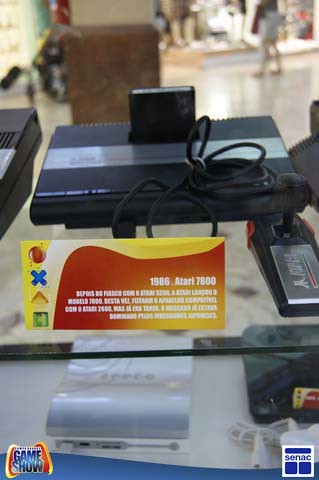This photograph appears to be from a second-hand store or perhaps a museum display. Centered prominently in the image is a vintage Atari 7800 console, identifiable by a stylized sign in the foreground that reads "1986 Atari 7800." The sign features a yellow and orange background with white text and includes a brief, four-line description written in what seems to be Italian, though the full text is difficult to discern from this distance. The Atari system is situated on a glass shelf, with cables coiled around it.

The background reveals a wooden bookcase-like structure and several people strolling, suggesting a mall-like environment. On the shelf beneath the Atari, there are a couple of other video game systems: one is white with some indistinguishable text, and the other is black. In the bottom left corner, there's a logo on the same yellow and orange backdrop as the Atari sign, displaying the words "Game Show" in a bluish font. The bottom right corner features another logo for "CENAC," designed in royal blue and white.